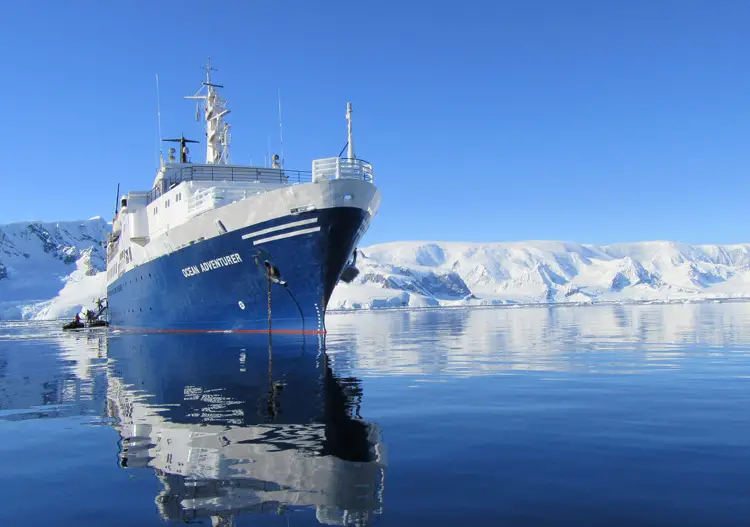In this serene scene, calm waters reflect a pristine blue sky with impeccable clarity, creating an almost mirror-like surface. The centerpiece of the image is the large vessel, Ocean Adventurer, prominently featuring its name in white letters on its blue lower half. The ship boasts a blue hull with a white trim at the top, ascending into multi-story white structures complete with radars, antennas, and communication equipment. A black railing borders the upper deck, designed for observation.

The anchor is deployed at the front of the ship, detailed and visible as it descends into the tranquil water. In the background, a snowy, icy landscape stretches out, mixing with patches of barren earth and rocky formations. This rugged terrain appears flat-topped with jagged sides, predominantly white from the snow but interspersed with dark gray rock. The water’s clarity allows the ship’s reflection to be seen vividly, enhancing the overall scene's tranquility and stark beauty.